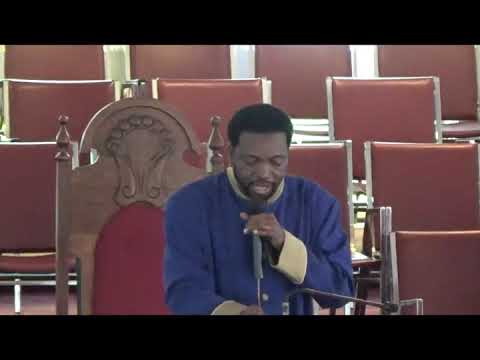The image appears to be a low-resolution screenshot from a video, depicting a religious event. Central in the frame is an African-American man with a short, slightly poofy afro and a light beard, who seems to be delivering a sermon or prayer. He is holding a microphone with his left hand and looking down, possibly reading from a passage. His attire is a blue jacket with beige-yellow cuffs and collar. Behind him, there's an ornate brown wooden chair with an arched top and decorative elements resembling canopy bed posts, suggesting a church setting. Further back, rows of cushioned, reddish-brown seats, akin to choir pews, are lined up, framed by an arched, red background reminiscent of stained glass windows. The image is flanked by black stripes at the top and bottom, emphasizing the central scene.